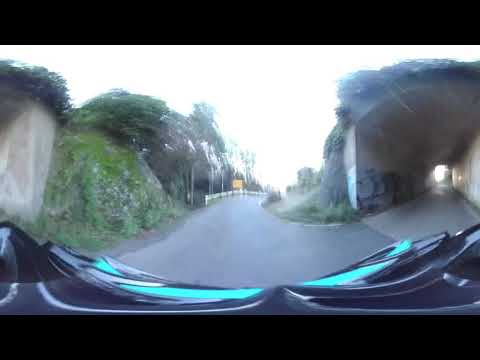The image captures a scene from the perspective of a person in a vehicle, possibly a car or motorcycle, driving on a wide, paved road under a bright gray sky. The road approaches a fork, with one path curving to the right towards a tunnel partially covered with ivy and greenery, including trees and plants. The tunnel's entrance and interior feature visible graffiti. A yellow street sign is seen far ahead, though its details are indiscernible. On either side of the curved road, white fencing lines the path. To the left, vibrant green bushes are warped, giving a melting appearance, possibly due to special camera effects or virtual reality manipulation, leading to a block-like structure that could be the start of another tunnel. Overall, the image presents a warped, somewhat blurred outdoor daytime scene with elements of nature and urban infrastructure blending together.